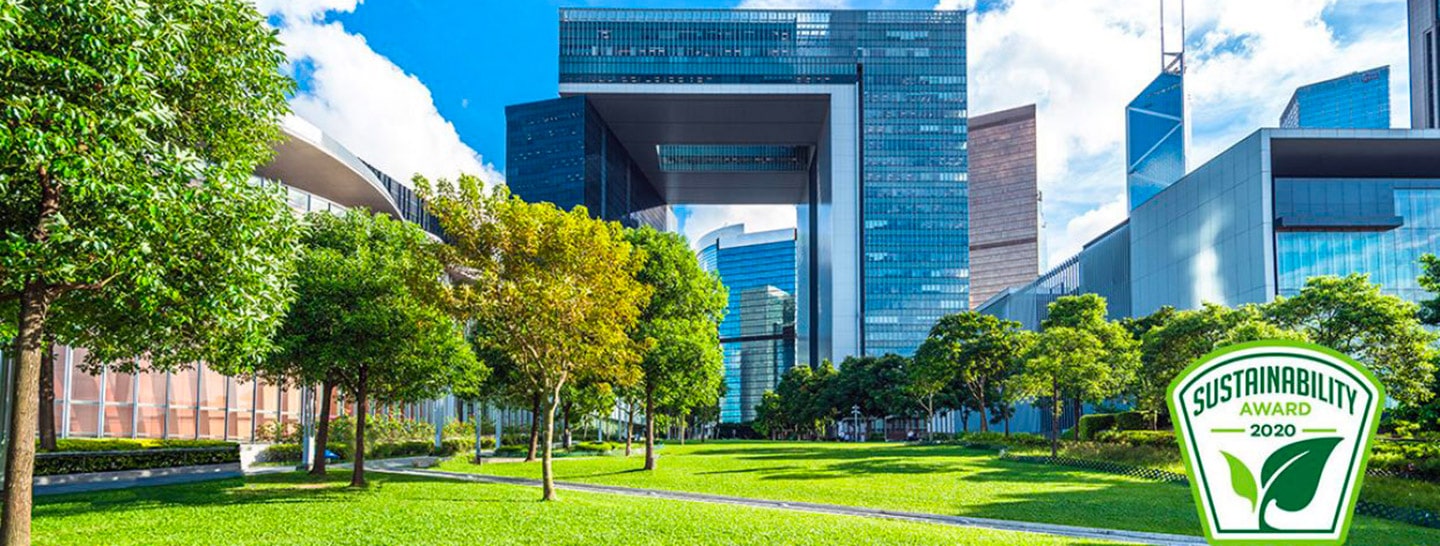The image features a narrow, long photograph depicting a vibrant park scene with modern-style skyscrapers in the background. In the center background, a distinctive L-shaped skyscraper, possibly capital L-shaped and partially see-through, creates a cantilever effect that divides the building. A mixture of blue and grey steel and glass structures dominate the skyline, highlighting contemporary architecture. The photograph captures a clear, bright day with some scattered clouds.

In the foreground, a green, well-maintained lawn takes up most of the space, bordered by deciduous trees with predominantly green foliage, some starting to turn yellow. Walkways lined with trees cut through the lawn, creating a structured but natural scene. On the left side of the image, another building partially hidden by trees features expansive windows that reflect the surrounding greenery.

On the right-hand side, a "Sustainability Award 2020" seal, complete with a stylized leaf drawing, indicates that the building or the overall property has been recognized for its sustainable design and practices.